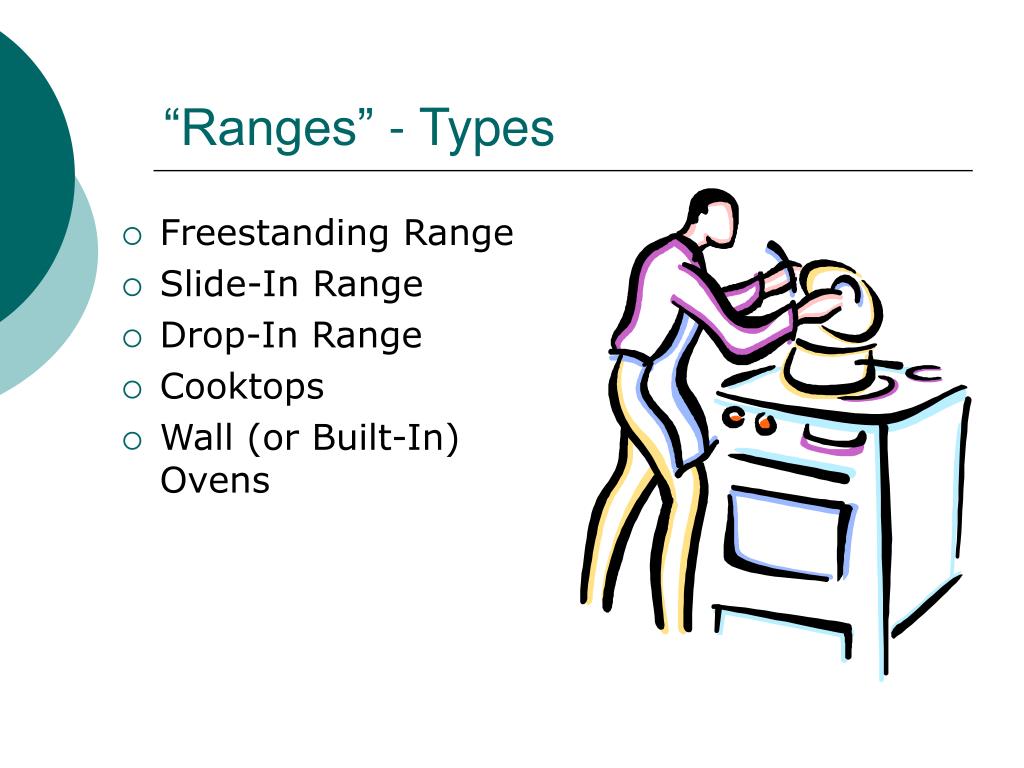The image resembles a PowerPoint slide set against a white background. In the upper left corner, decorative half-circle designs in dark and light blue add a touch of color. To the right, in a dark blue-green font, the text reads "Ranges - Types" beneath a thin dark gray line. Below this heading, bullet points list various types of ranges: Freestanding Range, Slide-In Range, Drop-In Range, Cooktops, and Wall or Built-In Ovens. On the right side of the image, there's a pencil sketch of a man cooking. The man is outlined wearing a purple shirt, brown or white pants, and a blue apron. His right hand holds up the lid of a pot, while his left hand stirs with a spoon. The pot sits on a stove range, depicted with a couple of burners, an oven, and an oven drawer. The illustration has a simple, sketched look, using minimalistic lines to convey the details.